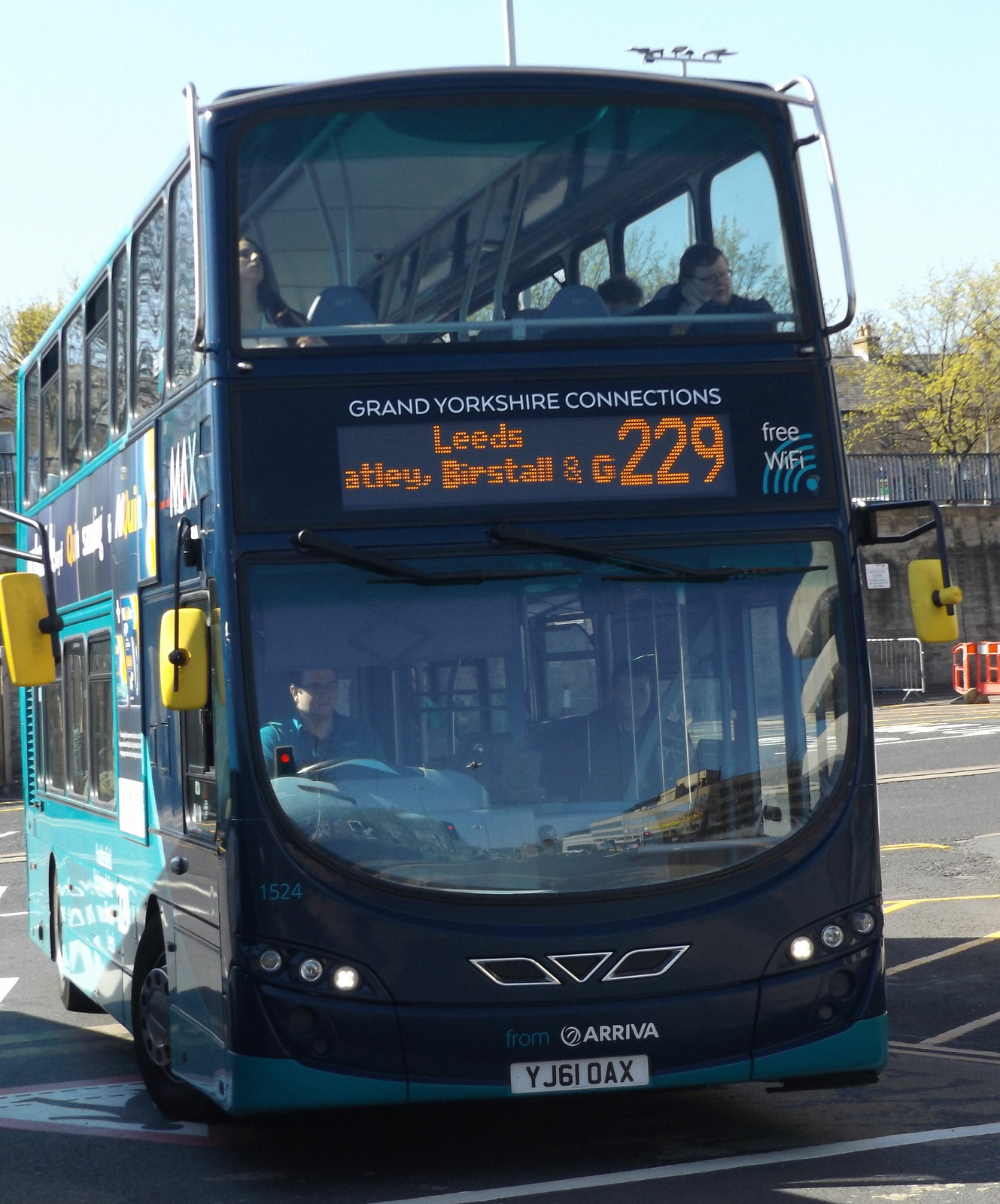This full-color daytime photograph captures a bustling street scene featuring a blue double-decker bus, which is an uncommon sight compared to the traditional red ones. The bus is partially shadowed, adding a dynamic contrast between the darkened front and the brightly lit rear. The driver is visible through a large windshield. Above him, passengers can be seen through another expansive window on the second level, making it clear that this vehicle accommodates two stories of seats.

The bus sports several windows along its sides and has distinctive yellow mirrors. It's adorned with turquoise and dark blue coloring, which transitions from a darker shade at the front to a lighter tone toward the back. The digital sign above the windshield reads "Grand Yorkshire Connections," flanked by "Leeds-Bertstow" and "G-229." Additional details on the sign include "Free Wi-Fi." Behind the bus, you can spot buildings possibly constructed from gray concrete, trees, a blue sky, as well as a roof and chimney. The pavement features yellow and white road striping, indicating a well-organized urban setting. The license plate reads YJ610AX, marked with "from Arriva." The varied light conditions, with the bus entering a shadowy area while the background remains bright, add depth to this vibrant street photograph.